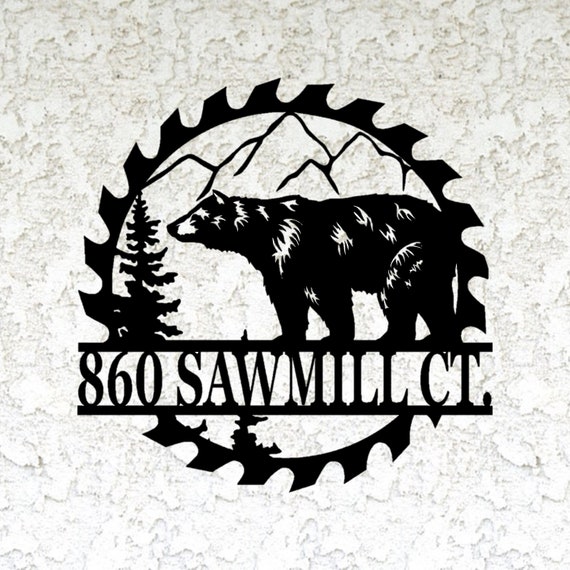The image is a detailed, black and white drawing resembling a logo, set against a heavily textured white background with a marbled or granite appearance. Dominating the center of the image is the black outline of a circular saw blade with prominently serrated edges. Inside this saw blade outline, there is a sketch of a mountain range at the top, rendered in black without shading. Below the mountains, a black bear facing left is depicted in profile with some black and white detailing, standing above a pine tree positioned to the left. Across the bottom of the saw blade is a banner with the text "860 Sawmill CT." The artwork is devoid of any other animals, people, or vehicles, and aside from the address, there are no additional inscriptions. This image could potentially represent a house number sign, but its exact purpose remains uncertain.